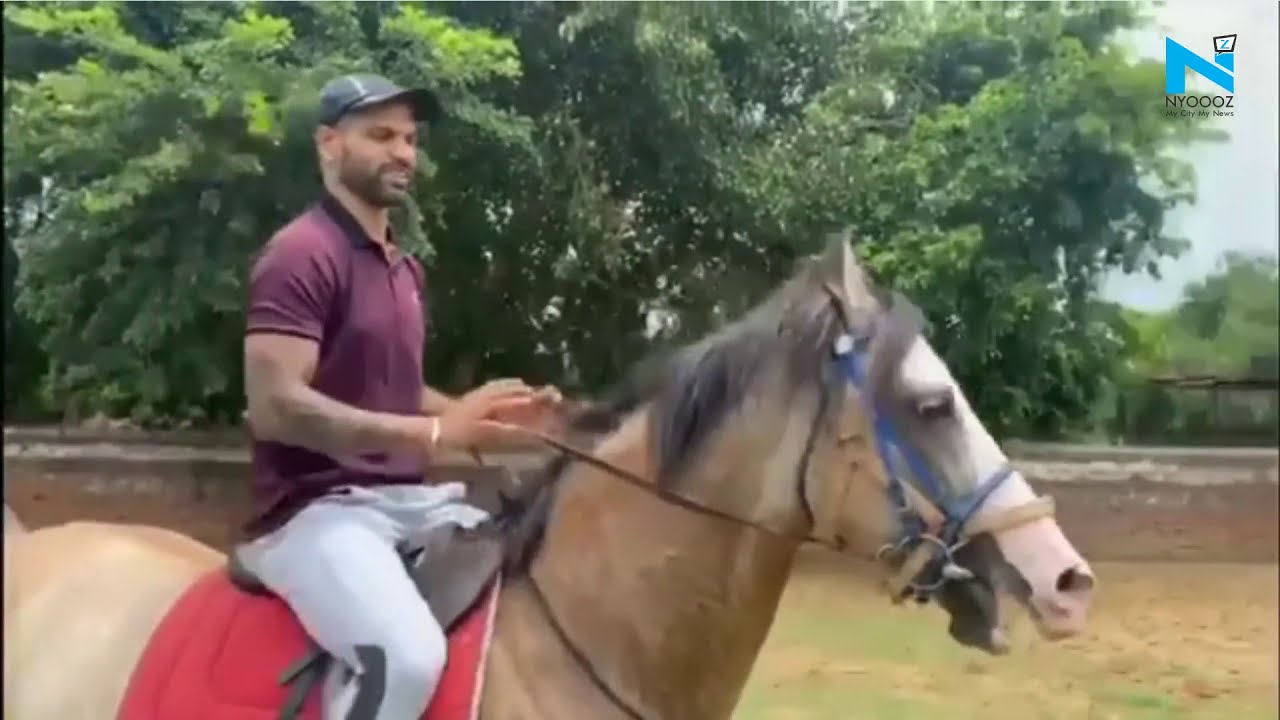The image depicts a young man, possibly in his late 30s or early 40s, who appears to be a horse jockey. He is riding a horse in the foreground of the photograph, with the duo moving towards the right or the three o'clock direction. The jockey, who has a light complexion that suggests he might be Middle Eastern or Caucasian, has a full or light beard and a mustache. He dons a dark-colored baseball cap, a purple short-sleeved collared shirt, and white pants—although one account mentions gray pants. 

The jockey holds the reins at a 90-degree angle as he rides a beige or pale palomino-colored horse with a charcoal gray or black mane and a white muzzle. The horse sports a red saddle and a dark blue or purple bridle. The background features a tree line with bright green leaves occupying the top two-thirds of the image, while the ground below, though grassy, appears sparsely populated and somewhat brownish. There is text in the upper right-hand corner of the image, featuring a stylized "N" or possibly a "Z" followed by "NY" or "N-Y-0," indicating a possible New York connection. The overall scene suggests a tranquil training session in an open field.